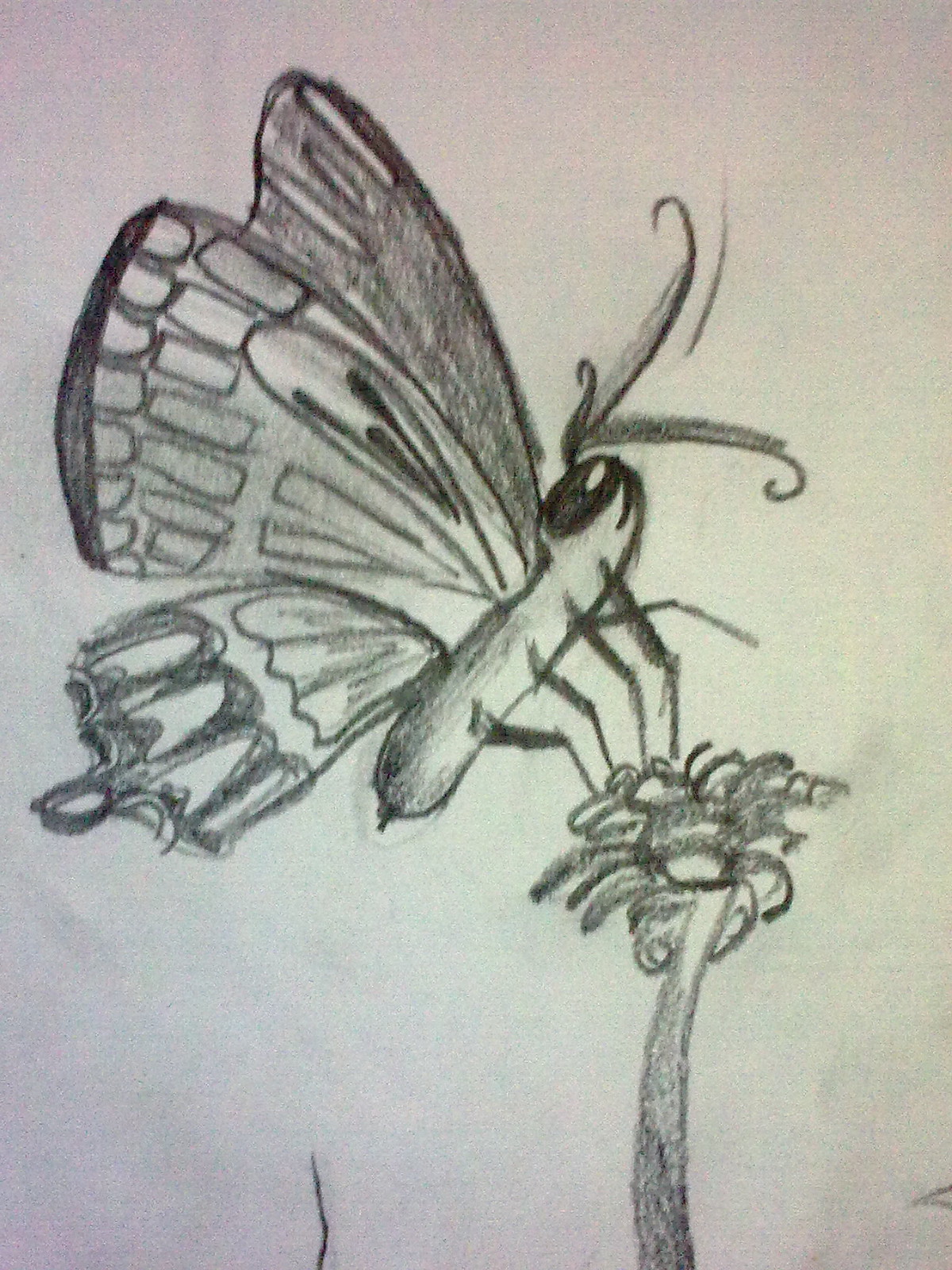This is a meticulously detailed pencil or crayon drawing rendered on a piece of slightly grayish paper. Dominating the artwork is a large butterfly positioned towards the upper and central portion of the image. The butterfly, characterized by its intricately designed wings, sits atop a flower with a long stalk emerging from the bottom right corner. Facing upward towards the top right corner, the butterfly's body resembles the shape of a hot dog, with long antennae extending from its head. It has four stick-like legs that delicately perch on the flower. The butterfly's wings are striking, with one section of the front wing shaded in gray, while the remaining areas feature intricate, uncolored outlines of various patterns. The flower itself is simple yet elegant, with several petals surrounding its top. The entire composition is crafted in grayscale, giving it a cohesive and subtle monochromatic appearance.